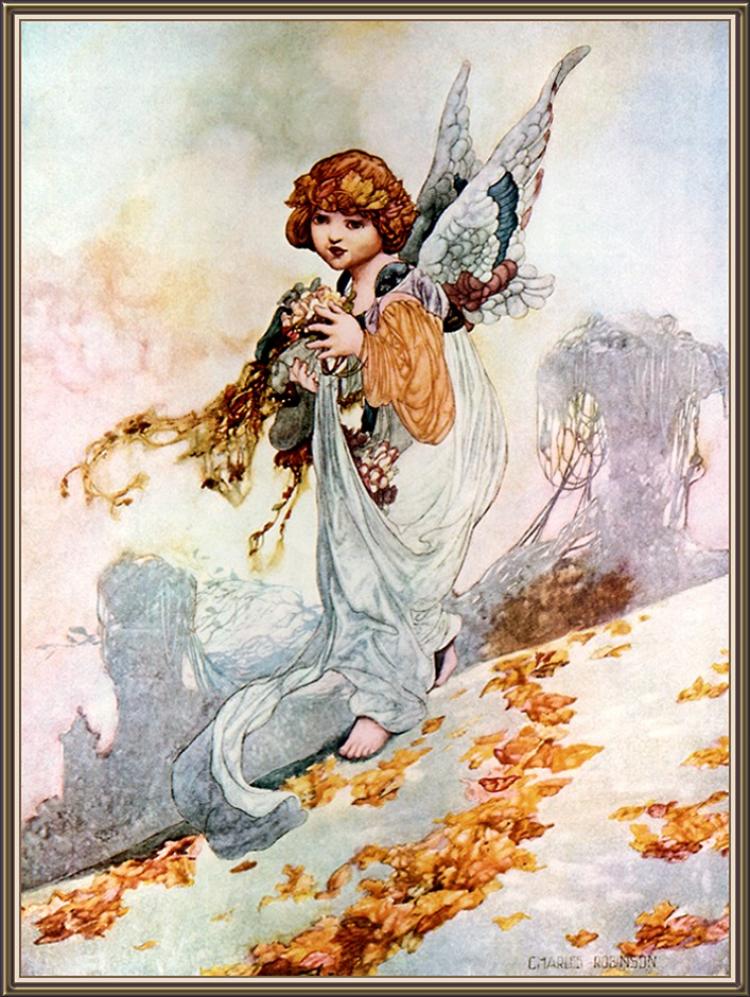In the image, there is a painting of a child angel standing on a slope or hillside covered with scatterings of orange and brown leaves. The angel is adorned with white wings that taper into shades of red, blue, and gold at the tips, and is wearing a flowing white robe along with a golden tunic. The angel's deep red hair is adorned with a floral hairpiece or a garland made of leaves, adding a touch of green. In one hand, the angel clutches a bundle of flowers or wheat-like foliage, which is also draped with an orange cloth. The background is predominantly a soft, light blue and white, giving a serene and ethereal atmosphere, with string-like trees adding subtle intricate details. The child angel is noticeably barefoot, with no footwear covering their feet. The overall tone of the artwork harmonizes with shades of white, gold, and autumnal hues, creating a delicate and peaceful scene.